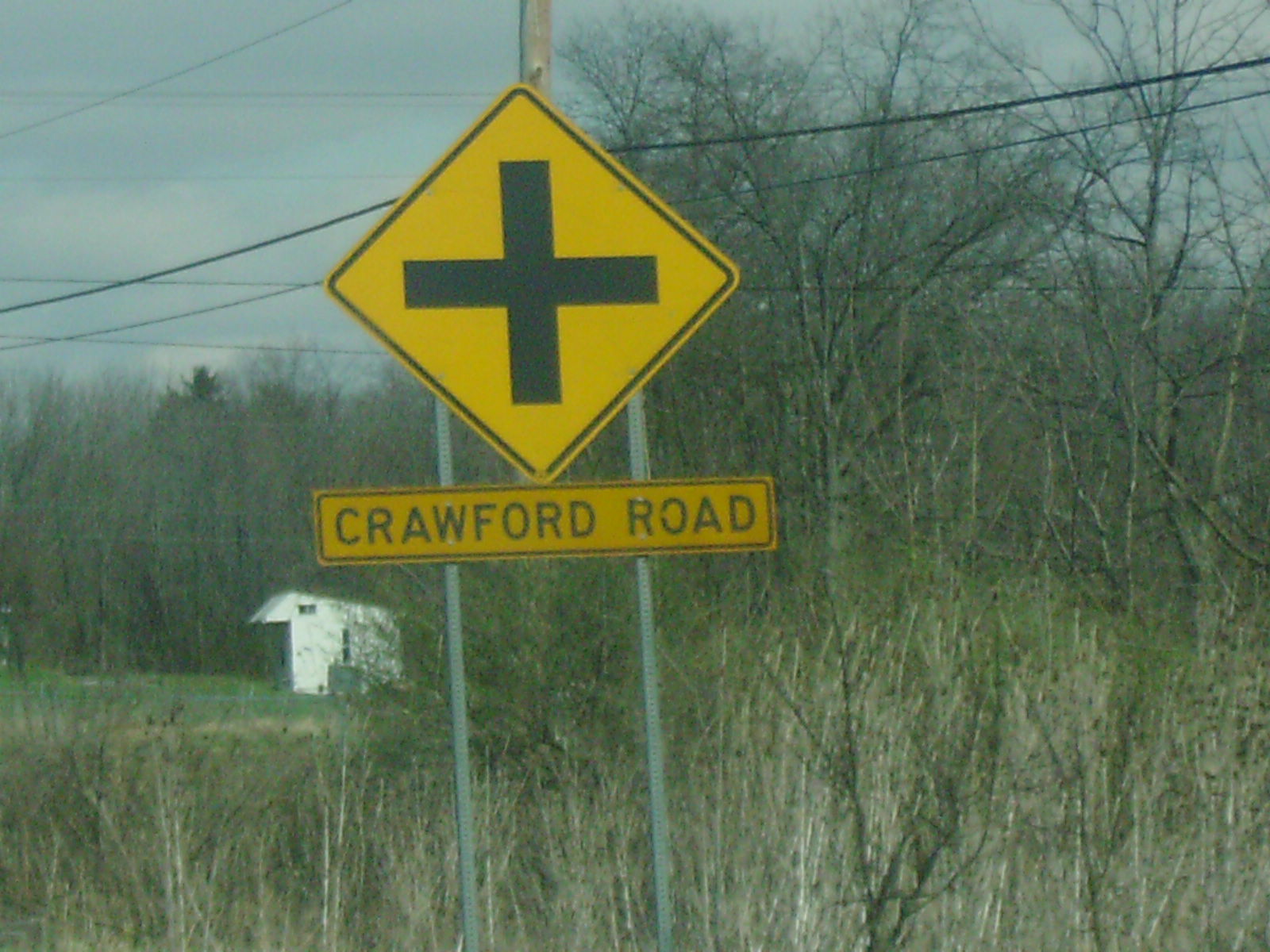In this photograph taken in a natural setting, we see an overgrown field of gray and brown grass, which stands tall and appears to be in a state of decay. In the distance, leafless brown trees add to the somber mood of the scene. The sky is a grayish-blue, overcast with clouds, casting a muted light over the landscape. To the back left, a small white building can be faintly seen, partially obscured by the encroaching grass. Dominating the foreground are two silver posts supporting street signs. The lower sign is yellow with a black border, bearing the name "Crawford Road" in black letters. Above it, a yellow diamond-shaped sign with a black border features a black cross, indicating an intersection ahead. The composition is dominated by the natural elements, with the signs providing the only hints of human presence.